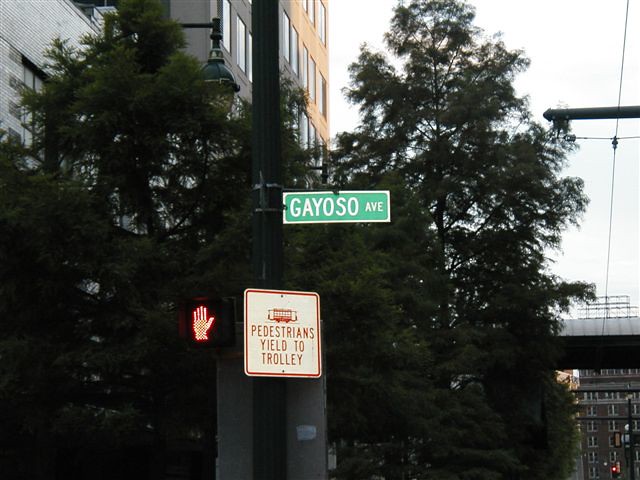The color photograph captures a quintessential American streetscape, prominently featuring a tall utility pole. Attached to the pole are two main signs: a green, oblong street sign with white lettering spelling out "G-A-Y-O-S-O-AVE" and a white sign marked with a red line and a tram icon, instructing "Pedestrians Yield to Trolley." An LED display adjacent to these signs is currently lit with a red hand, indicating no walking. In the background, the scene expands with a tall, brown brick building featuring many windows, some of which are long and triangular. Lush trees and a network of utility wires crisscrossing the image provide additional context. On the far right, part of a bridge is visible above the apartment blocks, contributing to the layered urban view. There are no vehicles, people, animals, or flowers present, offering a focused look at the signage and urban landscape.